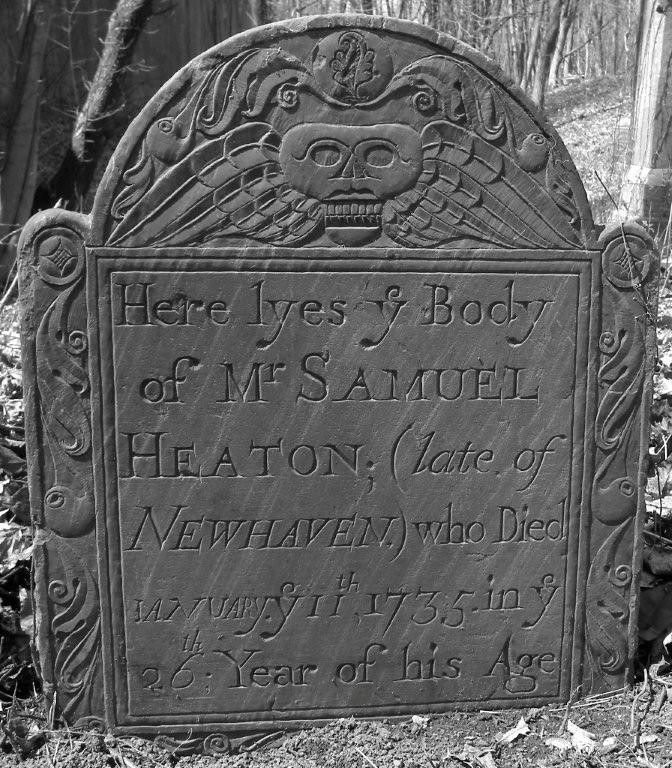This black-and-white photograph captures an old tombstone, seemingly centuries old, possibly made of weathered gray stone. The cemetery setting is marked by a backdrop of leafless trees and scattered undergrowth, suggesting an autumn or winter season. The tombstone, adorned with intricate designs, features a bird's head on the right and left sides of its arched top. Below this, a circular motif encapsulates a leaf, followed by a prominent human skull with angel wings on either side. Further down, there is a chisel detail near the base. The stone's inscription reads, "Here lies the body of Mr. Samuel Heaton, late of New Haven, who died January 11th, 1735 in the 26th year of his age," with notable archaic spellings such as "lies" spelled as "lyes" and the stylized use of "Y" for "the." The foreground shows a mix of dirt and dried leaves, enhancing the scene's age and somber atmosphere.